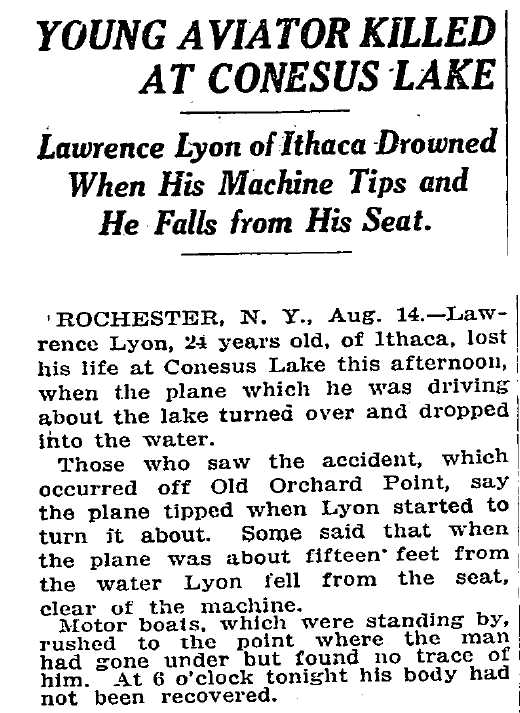The image depicts a grayscale cutout from an old newspaper, showcasing black text on a white background. The headline reads, "Young Aviator Killed at Conesus Lake." It reports the tragic incident involving Lawrence Leon, a 24-year-old from Ithaca, who drowned when his airplane tipped over, causing him to fall from his seat. The accident occurred at Conesus Lake, near Old Orchard Point, on the afternoon of August 14th in Rochester, New York. Eyewitnesses mentioned that the plane tipped when Leon attempted to turn it about 15 feet above the water. Despite the prompt efforts of motorboats rushing to the scene, no trace of Leon was found by 6 o'clock that evening when his body had still not been recovered.